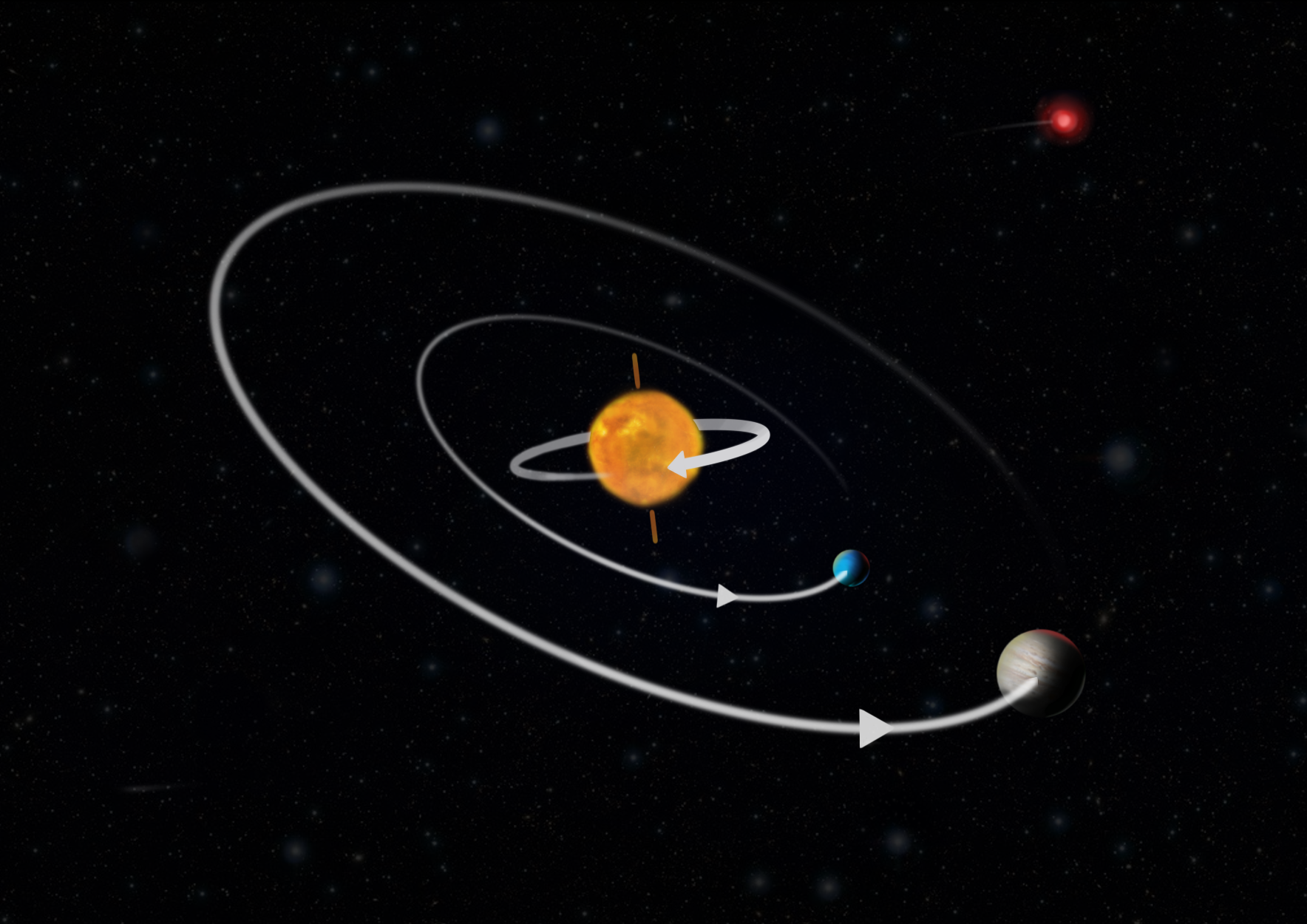This image is a detailed animated artwork of space. It features a black background dotted with faint white stars, enhancing the cosmic theme. In the center of the image is a large yellow-orange Sun. Two white arrows illustrate the motion around the Sun: one showing a clockwise rotation and the other depicting the Earth's counterclockwise orbit. A smaller white arrow indicates the Moon's counterclockwise path around the Earth. Additionally, the image includes a smaller blue planet identified as Earth, visually connected by the orbital arrows.

In the upper right corner, there is a small, shiny red light that stands out against the dark background. Scattered around the scene are tiny, faded light blue balls. Central to the composition are multiple white circles and arrows, with one large central circle featuring an arrowhead pointing towards a white-colored planet with stripes, and a similar smaller circle pointing towards the blue Earth-like planet.

Overall, the intricate diagram illustrates the rotational and orbital dynamics of the Sun, Earth, and Moon, highlighted by the use of arrows and circular paths, creating a comprehensive celestial display.